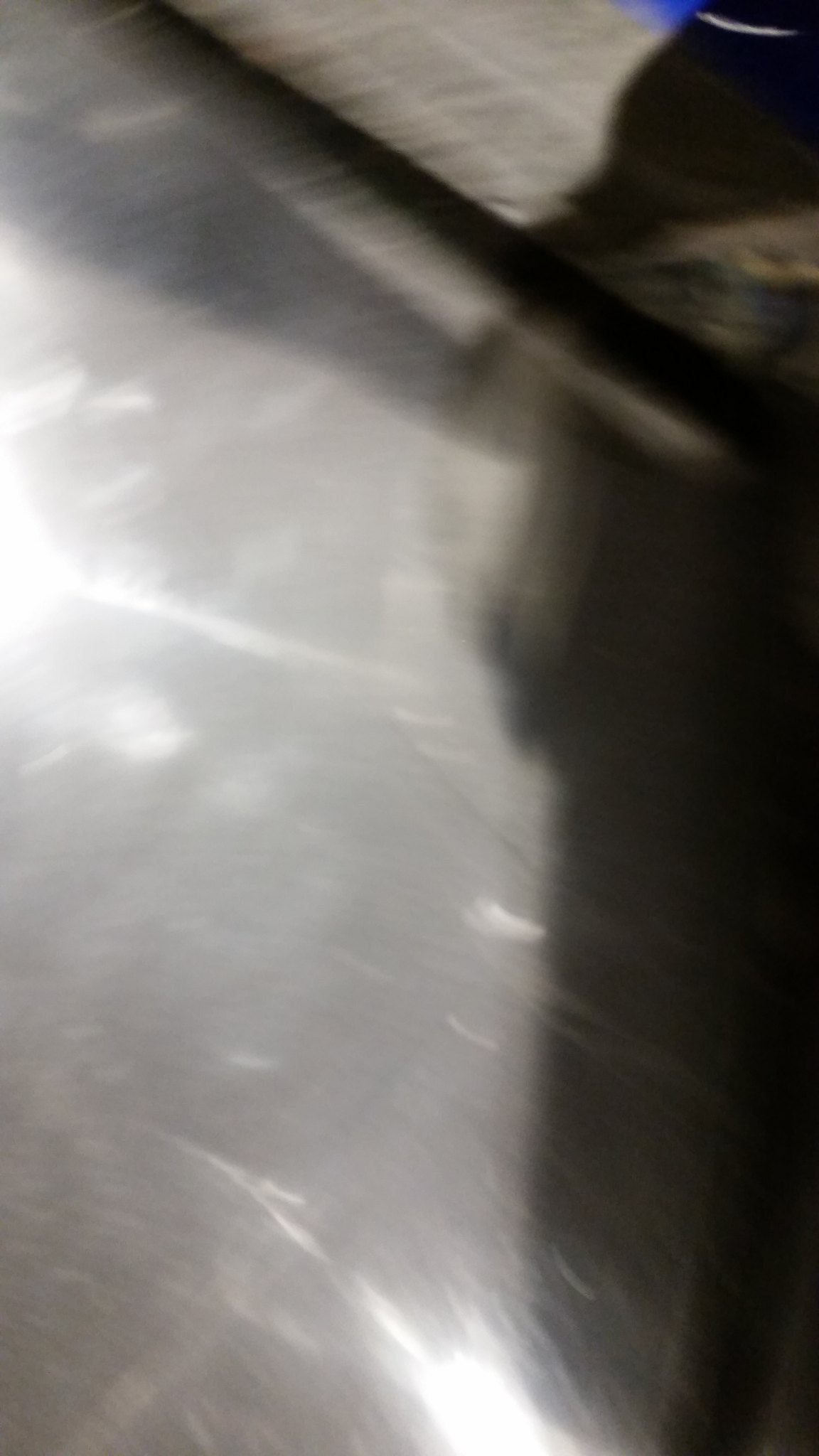This color photograph, taken outdoors, captures a scene featuring the side of a sidewalk and a portion of a road. The closest part of the image depicts the road, transitioning into a curved section that leads to the sidewalk. An indistinct object, standing on the sidewalk, casts a prominent shadow stretching across the road and reaching the bottom right-hand corner of the frame. Additionally, two reflective lights are visible—one positioned near the bottom center and the other midway up the left-hand side—adding a subtle glimmer to the scene. The blurriness of the image imparts a mysterious and somewhat ethereal quality to the depicted objects and their surroundings.